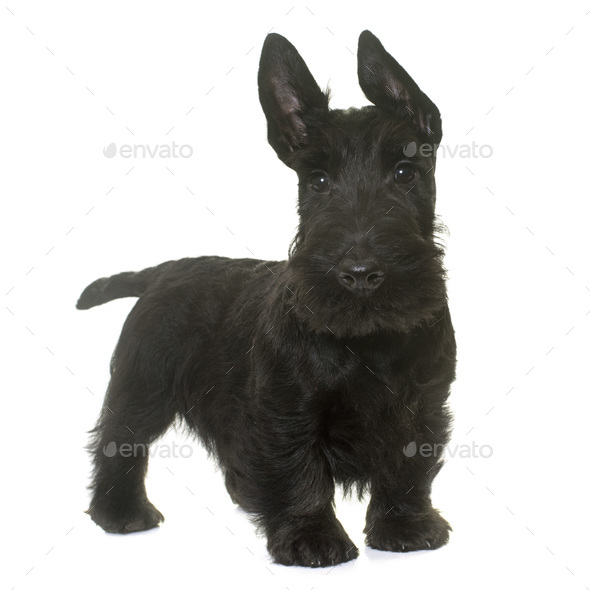The image features a small, alert, black dog with super furry, shiny black fur. Its ears, lighter pink on the inside but predominantly black, point straight up, giving it a strikingly alert appearance. The dog’s stubby tail sticks out, and it's standing on all fours, showcasing its petite size that could easily be mistaken for a rabbit. The vivid detail reveals its eyes, nose, legs, paws, and even nails. The dog stands against a stark, white background adorned with faint, gray "Envato" watermarks repeated four times in the left, right, bottom left, and bottom right corners, intersected by diagonal dotted lines. This watermark pattern suggests the image may be sourced from a digital platform, such as Google Images. Overall, the central focus remains the small black dog poised at attention, with the background elements subtly enhancing the stark contrast and highlighting the main subject.